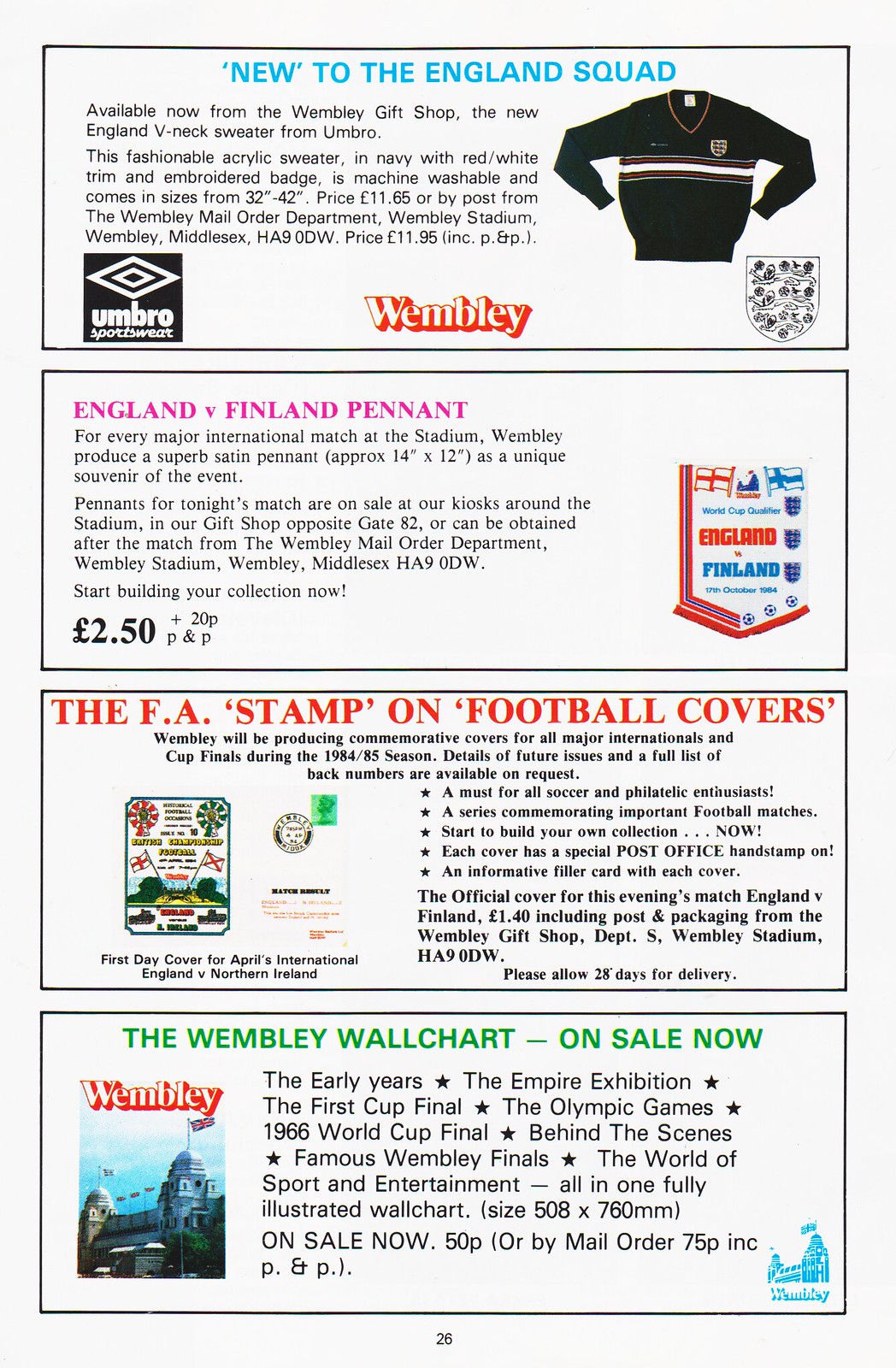The image is a series of four stacked rectangular advertisements on a light blue background, promoting various football accessories. The top rectangle features blue text on a white background stating, "New to the World." It highlights the "New England V-neck sweater from Umbro," with an image of the sweater to the right and the Umbro logo in a black square at the lower left corner. Below, the word "Wembley" is in red text accompanied by a crest and a sweater image on the right.

The second rectangle uses pink text reading, "England vs. Finland Pennant." It mentions that Wembley produces a satin pennant as a unique souvenir for major international matches, with the pennant image showcased on the right and a price of 250.

The third rectangle features red text that says, "The FA Stamp on Football Covers." It describes Wembley's production of commemorative covers for all major internationals and cup finals during the 84-85 season, with an image of a cover on the left.

The final rectangle is titled "The Wembley Wall Chart on Sale Now" in green text. It includes a paragraph about the wall chart, displaying an image of it on the left, along with a photograph of a building and the Wembley logo.